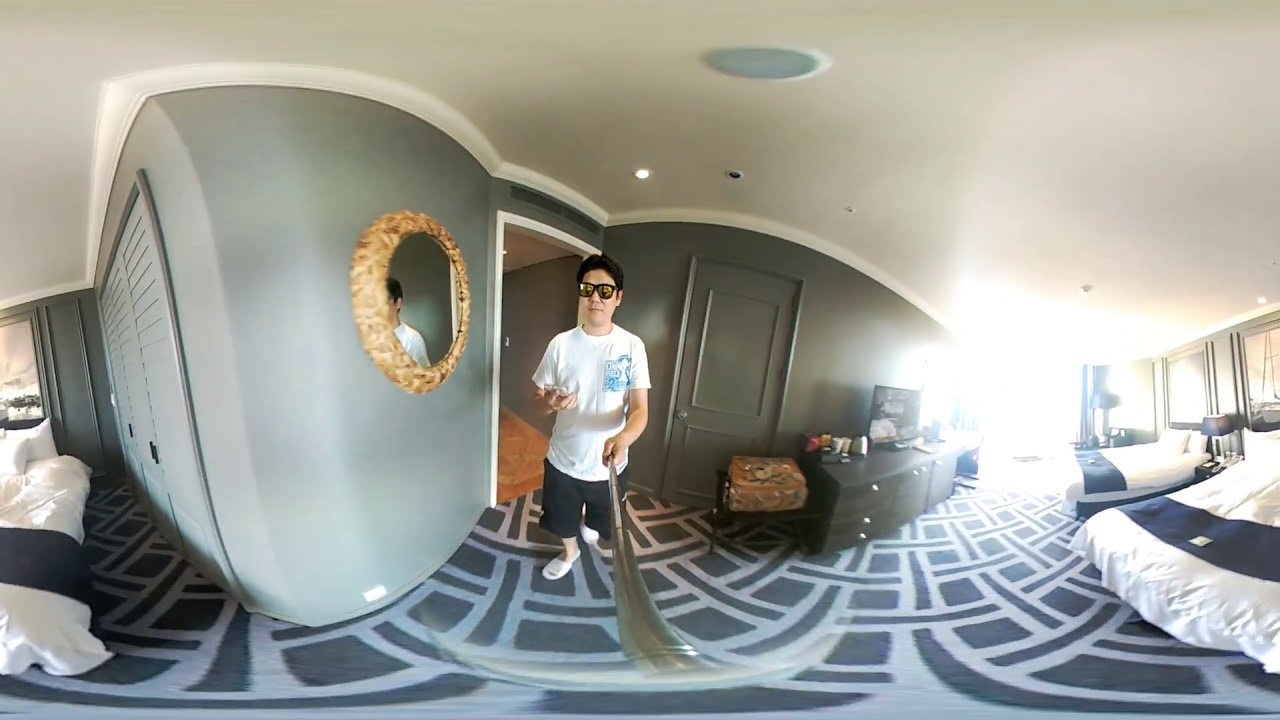The image shows a man, likely in his 20s, taking a selfie with a selfie stick indoors, possibly in a hotel room. He has short black hair and is wearing black-framed sunglasses, a white short-sleeved t-shirt with a blue design, black shorts, and white flip-flops. The room is furnished with two queen-sized beds with white sheets and decorative blue bands, arranged on the right side. There appears to be a partial view of another bed on the left. The floor features a patterned rug in light and dark blue hues. The walls are gray with white trim, and the ceiling is white with recessed lighting. A dark brown dresser with a small TV on top is situated against one wall, and a round, gold-colored mirror hangs nearby. The overall layout and details of the room suggest it is a hotel room.